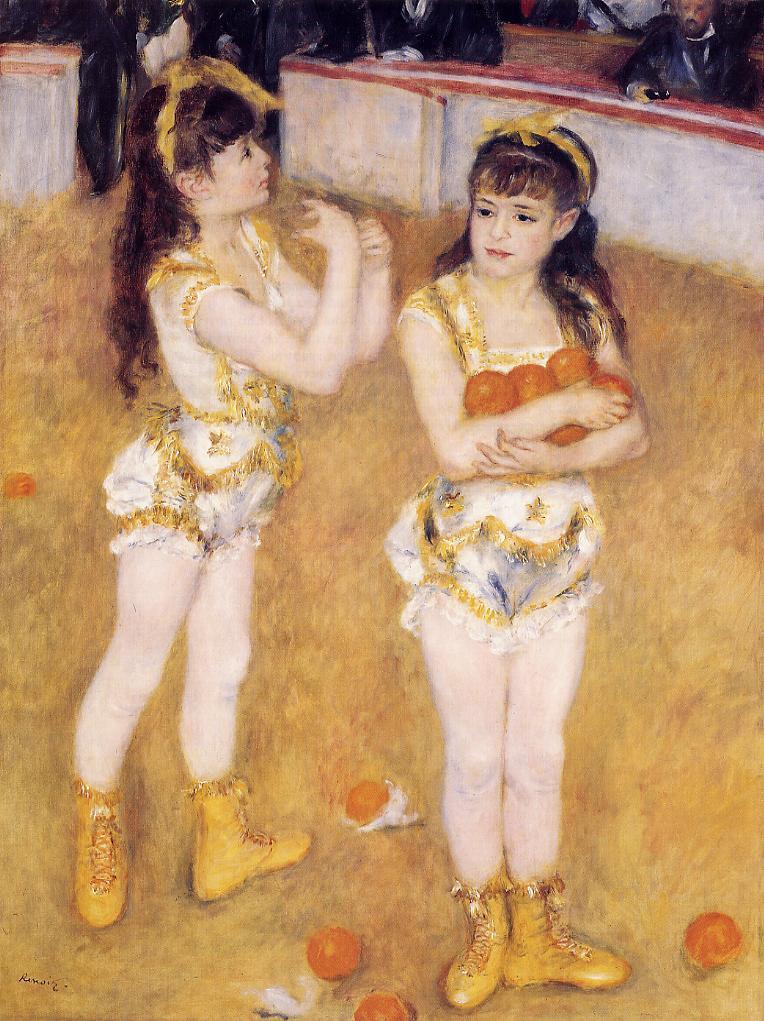The painting portrays a nostalgic circus scene featuring two young girls, likely twins around 10-12 years old, dressed in elaborate, early 1900s circus uniforms. They stand on a grassy, yellow-hued arena floor bordered by a low, circular wall painted white with a red top. The central focus is the girls, both wearing white unitards adorned with gold frills, yellow knee-high boots, and yellow ribbon headbands in their long brown hair, accentuated by matching bangs. 

The girl on the right is holding several orangish-red balls, possibly tomatoes or oranges, cradling them in her crossed arms. She looks toward the lower left side of the image with a calm or smirking expression. The girl on the left, gesturing upwards with her arms bent and hands open as if ready to catch something, faces towards the right side of the scene. Both girls' poses suggest a lively performance or act. Scattered around them are a few loose balls, adding to the performance atmosphere. 

In the background, a man sits against the circular wall, his right arm resting on it, while painted figures of men seem to observe the scene, enhancing the circus ambiance. The dominant colors in the painting are orange, yellow, white, and black, contributing to the vibrant and dynamic feel of this captivating moment from a bygone era.